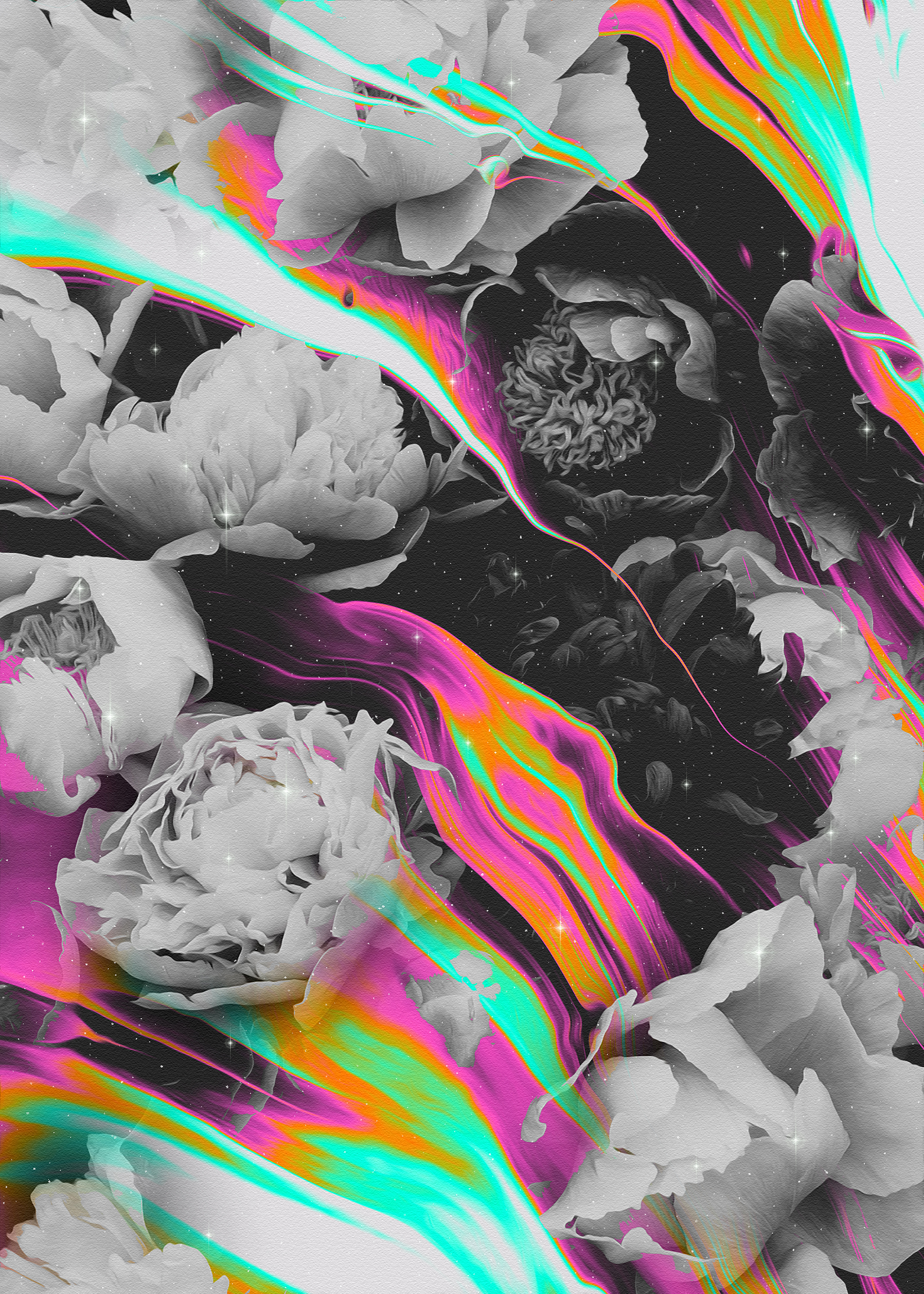The image presents a surreal digital artwork blending elements of photography and painting. It features an intricate arrangement of flowers, predominantly peonies and roses, rendered in black and white. These flowers, varying from fully bloomed to partially closed, are occasionally semi-transparent, giving a dreamy aura. Dominating the composition are vibrant, neon-like streaks of turquoise, white, gold, green, purple, and orange, which weave through the flowers in wave patterns, somewhat resembling rainbow-colored streams. These waves are semi-transparent too, allowing glimpses of an underlying black night sky replete with twinkling white stars and distant galaxies. Some flowers and colorful streaks appear sporadically concentrated in certain areas, especially the bottom half and corners of the image, enhancing the mystical ambiance. Central to the artwork is an unusual bloom with petals reminiscent of spaghetti noodles, adding a touch of abstract whimsy. The overall effect is a mesmerizing blend of natural and cosmic elements, creating a captivating visual interplay between the ordinary and the fantastical.